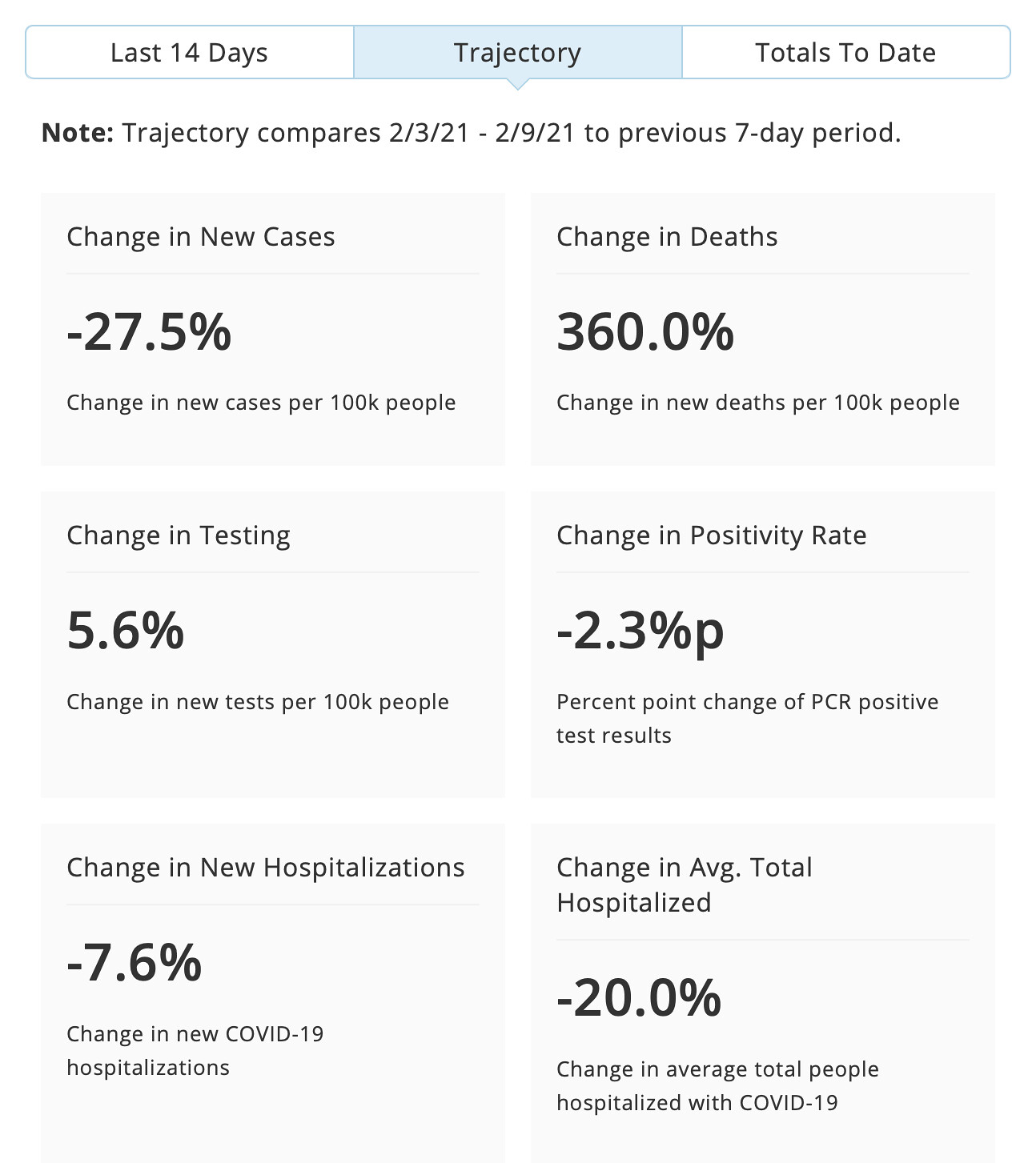This image displays a document detailing COVID-19 metrics from a hospital's activities in February 2021. The heading at the top reads "Trajectory," highlighted in blue against a light background, categorizing the data beneath it. It states, "Last 14 days trajectory and totals to date," followed by a note explaining, "Trajectory compares 2/3/21 to 2/9/21 to the previous seven-day period." The document is divided into two columns, each with several rows presenting percentages representing changes in key COVID-related statistics. 

Key metrics include:
- Change in new cases, marking a decrease of 27.5%.
- Change in deaths, indicating an increase of 360%.
- Change in testing, showing an increase of 5.6%.
- Change in positivity rate, down by 2.3%.
- Change in new hospitalizations, decreased by 7.6%.
- Change in average total hospitalized, which dropped by 20%.

Each category specifies whether the change is per 100,000 people or as a percentage point change, with supplementary information clarifying detailed statistics like PCR positive test results and COVID-19 hospitalizations.